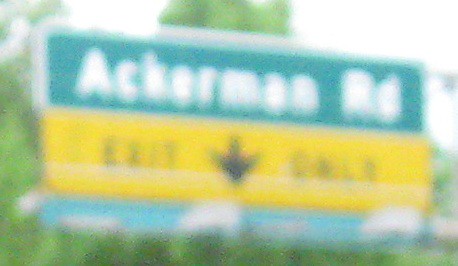The image depicts a green road sign that appears to read "Ackerman Road," although the exact text is difficult to confirm due to the low quality and blurriness of the photo. The sign is designed with a white outline and stroke. Below the main text, there is a yellow band that reads "EXIT ONLY" in black letters, accompanied by a black arrow pointing downward. In the background, there are visible trees under a blue sky, adding to the overall scene.